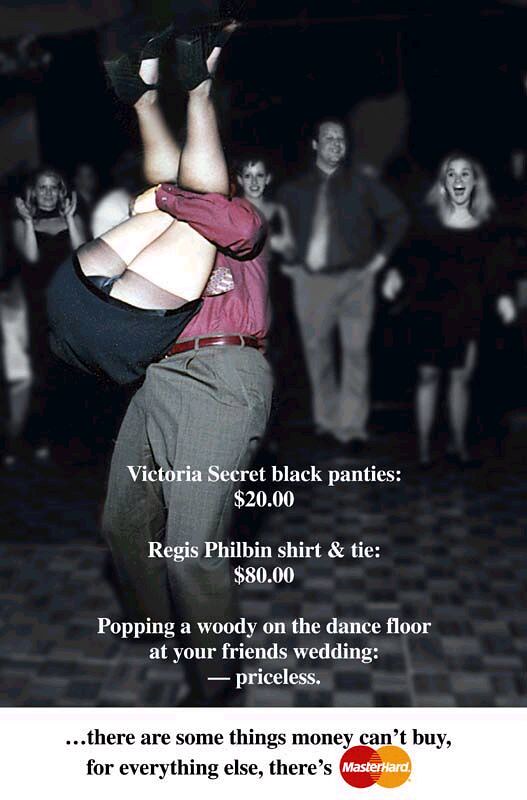In the foreground of this humorous advertisement, a man wearing gray pants and a red (burgundy) shirt is seen flipping a woman in a black dress with platform heels and black panties, revealing a bit of her underwear. The woman's face is not visible, and the man appears to have a bulge in the front of his pants. The backdrop is a checkered dance floor at a wedding, with several onlookers in the background smiling, clapping, and cheering. The photo is overlaid with humorous text: "Victoria's Secret black panties, $20. Regis Philbin shirt and tie, $80. Popping a woody on the dance floor at your friend's wedding, priceless." Below, the iconic tagline reads, "There are some things money can't buy. For everything else, there's MasterCard," accompanied by the MasterCard logo featuring red and yellow circles with overlapping white text.